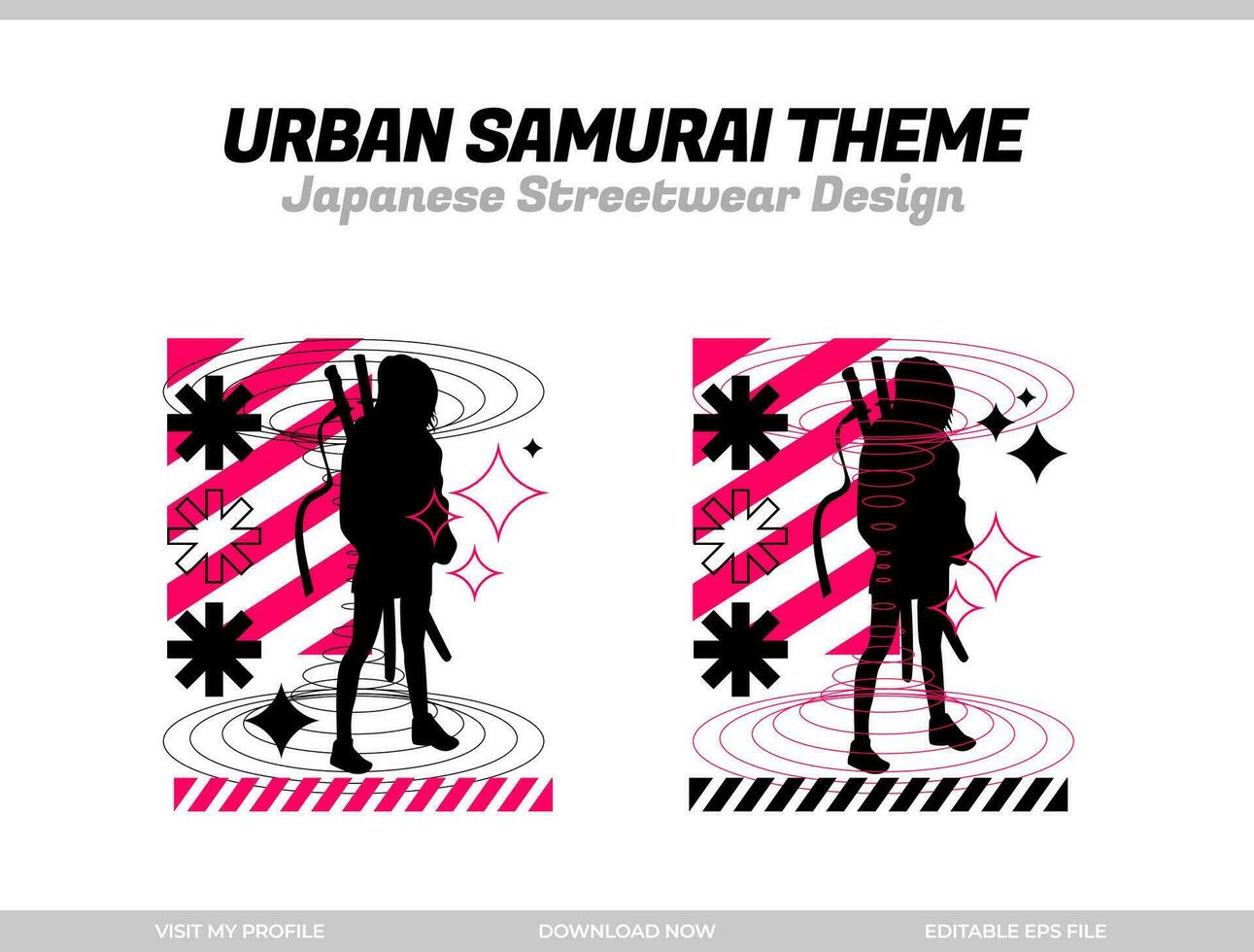The image features a stylized silhouette of a ninja with two short samurai swords on its back, set against a white background. At the top of the image, "URBAN SAMURAI THEME" is written in bold black font, with "Japanese streetwear design" in smaller gray font beneath it. There are two gray horizontal bars framing the top and bottom of the picture. The bottom gray bar contains three labels: "Visit My Profile," "Download Now," and "Editable EPS File," all in white text. 

The image is divided into two side-by-side sections featuring similar yet distinct designs. Both sections display a central ninja figure and sets of decorative red lines, black asterisks, and white asterisks on the left side. On the left image, there are vertical red and white lines at the bottom, while on the right, they are black and white. Both images also feature various stars and diamonds in black and pink, positioned differently on each side. The left image has pink diagonal lines, while the right one has similar lines but in black. Above and below the ninja silhouette, there are black circles in the left image and pink circles in the right image, adding to the urban aesthetic.